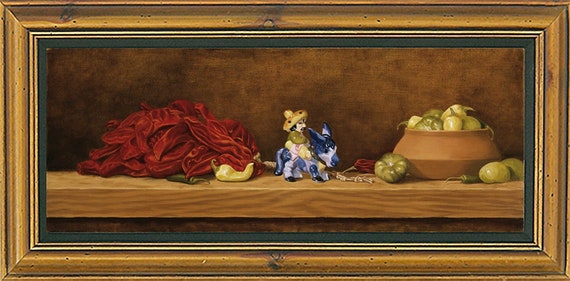This detailed still life oil painting, set against a brown wall, is housed within a gold-toned wooden frame featuring a green mat. The scene is meticulously arranged on a light brown wooden shelf. On the left side of the composition, there is a visually striking pile of dried red chilies, accented by one yellow chili and one green jalapeño pepper. Dominating the central area is a ceramic figurine—a blue and white donkey with a Mexican rider, wearing a sombrero and sporting a black mustache. On the right side, the shelf supports a tan bowl filled with green tomatillos, some of which spill out and rest on the shelf itself. Another dried red chili can be seen positioned behind the bowl. This classic still life painting captures a harmonious blend of colors and textures, reminiscent of traditional hotel art styles.